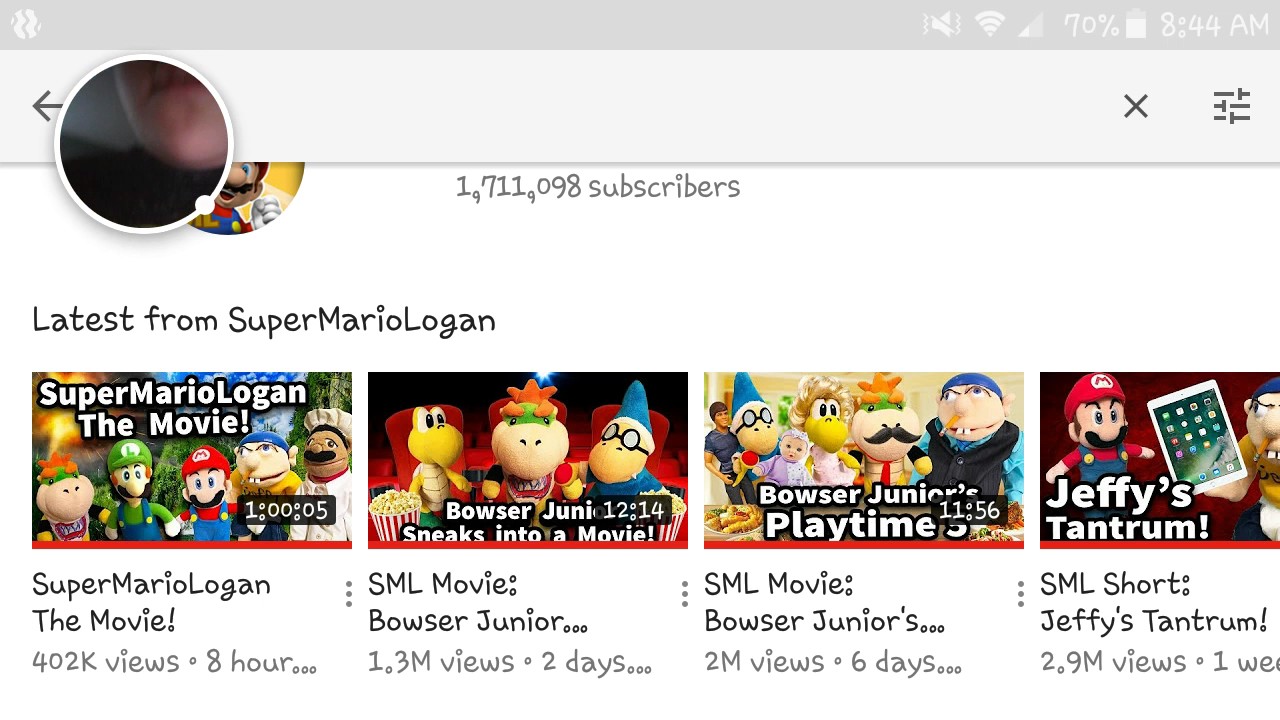**Detailed Caption:**

The screenshot has a clean white background and prominently features a profile picture displaying a person's chin. The top-right corner shows a battery icon at 70% and the time is 8:44 AM. To the left of the profile picture are a left arrow and a close (X) button. The page also displays a subscriber count of 1,711,098 subscribers for the popular YouTube channel "Super Mario Logan."

The first highlighted video is titled "Super Mario Logan The Movie" with a runtime of one hour and five seconds. It has garnered 402,000 views eight hours post-upload. 

The second video listed is titled "SML Movie: Bowser Junior..." with 1.3 million views over two days.

The third video is "SML Movie Browser Junior..." which has accumulated 2 million views in six days.

Lastly, there is an "SML Short: Jeffy's Tantrum" with 2.9 million views within one week.

Each thumbnail image associated with the videos provides a visual preview, further indicating that these titles are from the latest uploads by "Super Mario Logan."